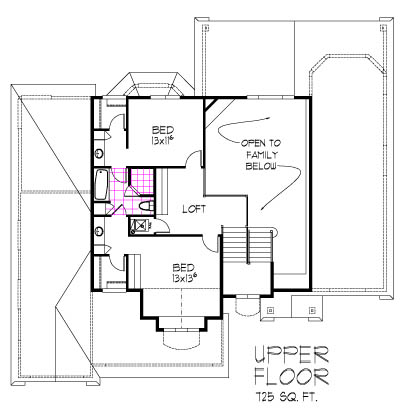The image showcases detailed architectural blueprints of a residential building. The focus is on the upper floor, which spans 725 square feet, as indicated at the bottom of the blueprint. This floor includes a 13 by 13 bedroom termed as "open to family below," suggesting a loft-like layout. An adjacent bathroom features a clearly drawn tub, highlighted in bold black lines. The blueprint also depicts a stairway descending to the lower floor, though the lower floor itself isn't labeled. The drawing is meticulously crafted on a stark white background, with sharp, precise lines delineating each feature. The central area, containing the bedroom and related spaces, is accentuated with thicker black outlines, drawing attention to these key components. The overall presentation is clean and uncluttered, without additional images or labels, underscoring the high-quality, professional nature of the blueprint.